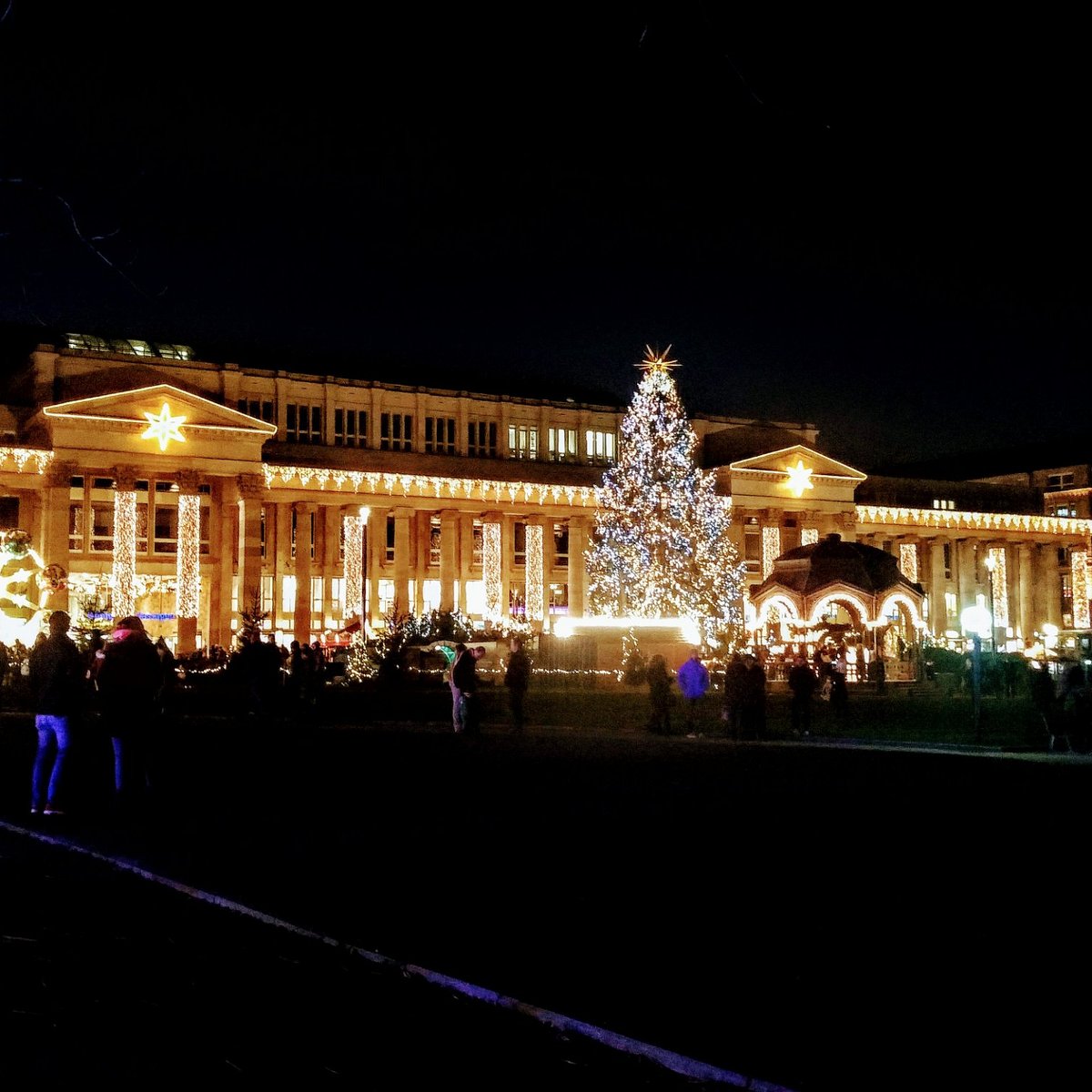In this nighttime scene, a long building, possibly a museum, stands out against a completely black sky and ground. The structure is illuminated with golden-yellow Christmas lights that wrap around its many pillars and roof. At the top corners of the building, two brightly lit snowflakes shine prominently. Central to the image is a large, fully lit Christmas tree adorned with a spiky gold star at its peak, adding to the festive atmosphere. Surrounding the tree and standing in front of the building, a crowd of people is visible, their presence highlighted by the glowing lights. The overall effect is a warm and inviting Christmas market scene, characterized by the brilliant illumination and the joyful assembly of visitors.